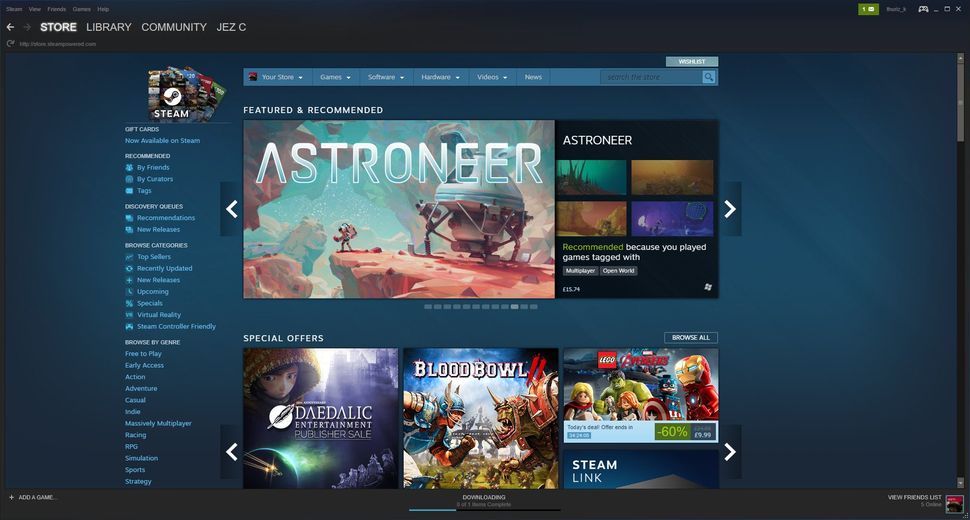This is a screenshot of the Steam website, a popular digital distribution platform for video games. The page showcases various recommendations and offers. The top of the page features a header with white text on a black background, displaying navigation options such as Store, Library, Community, Gift Cards, Recommended, and My Friends.

The main section of the website has light blue text on a dark blue background, and includes navigation links for Tags, Discovery Queues, Recommendations, New Releases, Browse Categories, Top Sellers, Regularly Updated, Upcoming Specials, and Virtual Reality.

A detailed browse-by-genre section at the bottom lists categories like Free to Play, Early Access, Action, and Adventure.

The central part of the image highlights a recommended game called "Astroneer," featuring an astronaut on the cliff of an alien planet with a spaceship in the background. This game is recommended because the user frequently plays multiplayer and open-world games.

Other featured content includes special offers on Daedalic Entertainment, a publisher sale, and an advertisement for "Blood Bowl," which depicts a ferocious man-beast and an armored human about to clash. Additionally, there's a Lego Avengers advertisement showcasing iconic characters like Iron Man, Captain America, and Hulk.